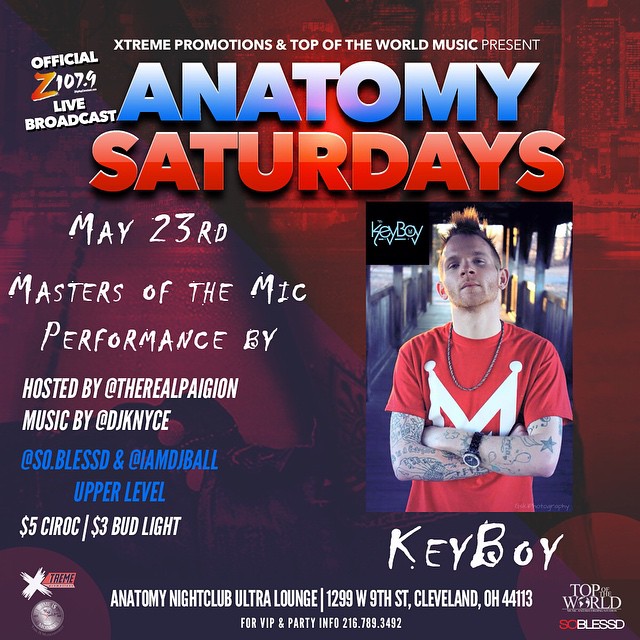The flyer, set against a bold red background, promotes an upcoming event featuring musician Key Boy, who sports a distinct look with tattoos covering his arms, a red short-sleeve shirt with a white logo, a watch, a necklace, and a mohawk dyed red. Key Boy stands confidently with his arms crossed. The event, titled "Masters of the Mic Performance," is hosted by The Real Pagan and features music by J-Sync. The event is scheduled for May 23rd, though the year is not specified. Additional text on the flyer includes mentions of VIP party information available at area code 216, a $5 entry fee, and $3 Bud Light specials. Notably, "Extreme Promotions and Top-of-the-World Music" and an official 107.9 live broadcast are highlighted, adding to the event's prestige. The location for this exciting event is Cleveland, Ohio.